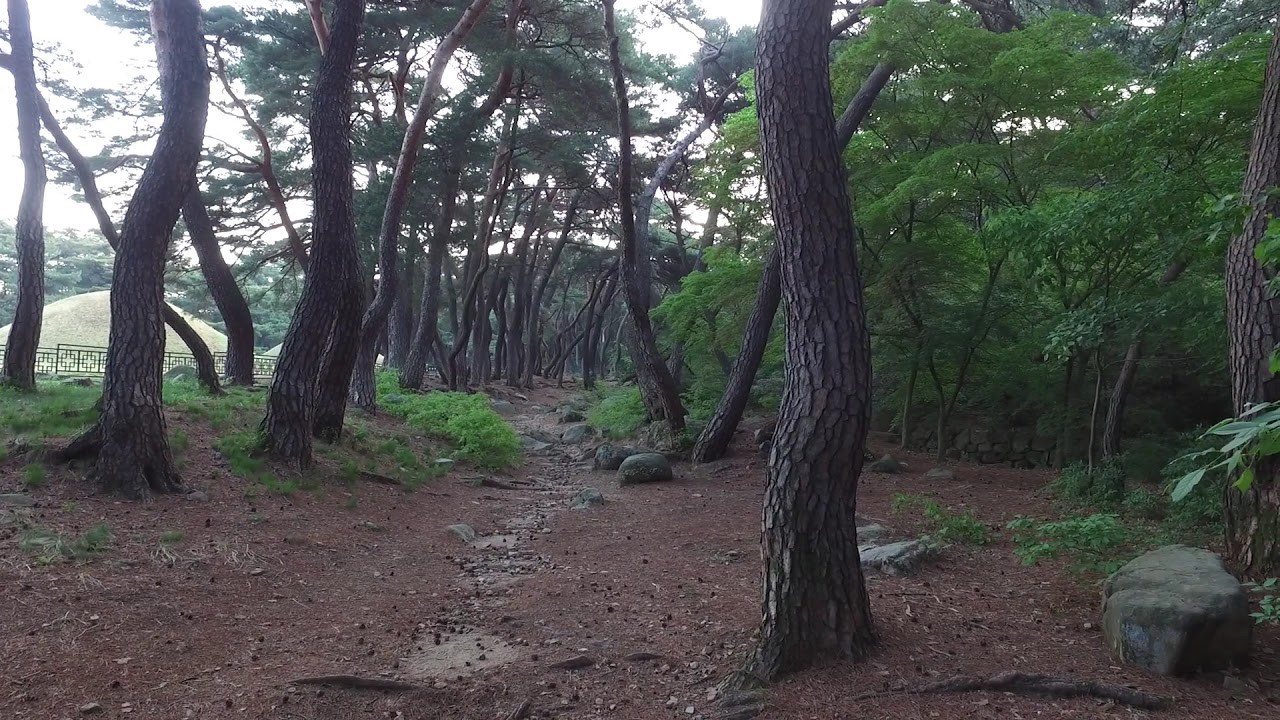In the image, a serene forest setting encompasses a narrow, muddy hiking trail interspersed with small and large rocks. The trunks of the abundant green-leaved trees display a distinctive scaled texture and an appealing crookedness, allowing glimpses of the bright, white sky above through their sparse foliage. The moist ground, hinting at recent drizzle or fog, contributes to the overall lush ambiance. On the left side of the trail, partially obscured by a line-patterned metal fence, stands a dome-shaped beige structure. This structure, perhaps an old mound or an architectural curiosity, contrasts with the verdant backdrop of trees that frame the entire scene. Scattered across the path and surrounding forest floor are a mix of concrete stepping stones, acorns, and natural debris, emphasizing the rustic and tranquil nature of this woodland area.